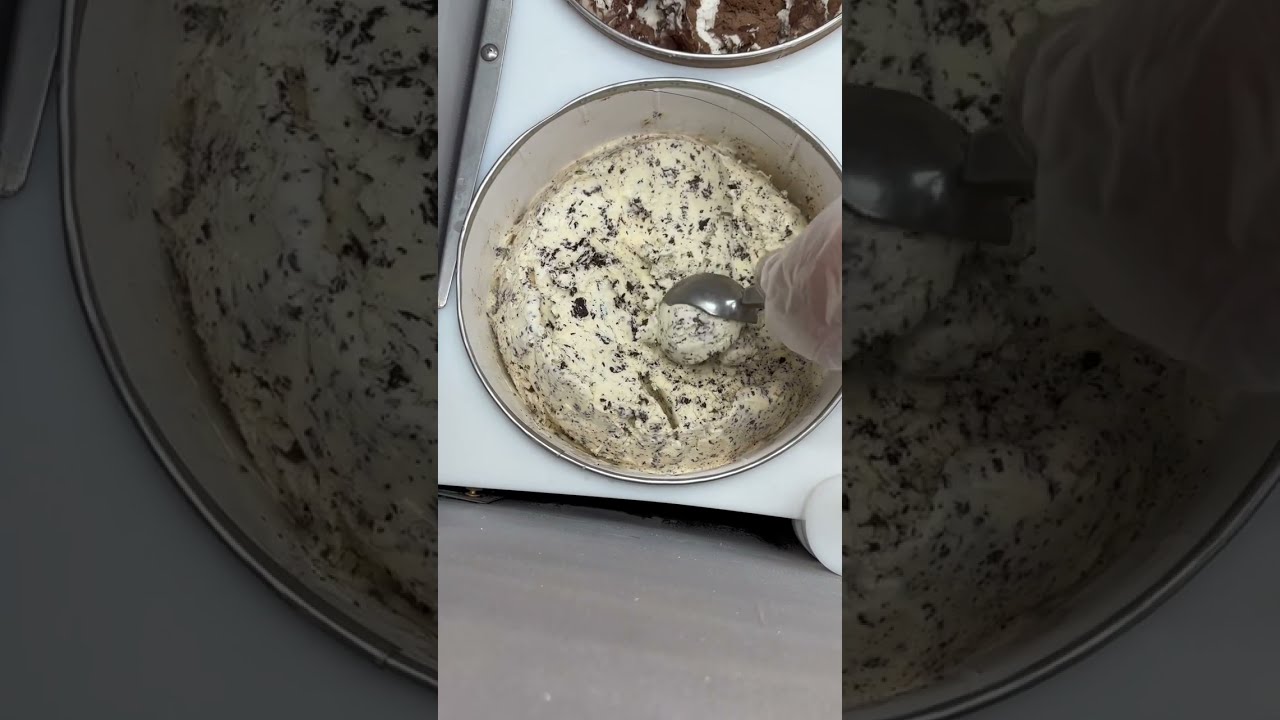In this detailed image, we see a person scooping what appears to be cookies and cream ice cream. The scene is set in an ice cream parlor, featuring a white case with recessed tubs of ice cream and a metal border around the top of each tub. The main ice cream tub being scooped from has a creamy white base with scattered black specks, indicative of the cookies and cream flavor. Above this tub, another flavor is visible, resembling rocky road, with a predominantly chocolate base interspersed with white swirls. The person scooping the ice cream is wearing a plastic glove and using a traditional silver ice cream scoop. The image is positioned horizontally in the center, bordered on the left and right by darker, blown-up segments of the same image, providing a zoomed-in effect on the ice cream tubs.